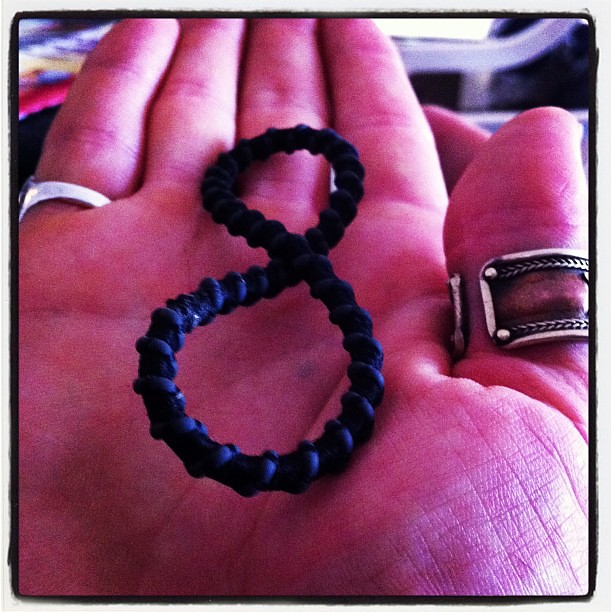In this square-format color photograph, a close-up shot reveals the detailed lines on the inner palm of what is likely a female hand. The image captures a black, ridged hair tie twisted into a figure-eight shape resting centrally in the person's outstretched, flat palm. Adjacent to the hair tie, the hand wears two distinct rings: a sterling silver pinky ring and a unique thumb ring, which appears to be a combination of brown and silver elements, possibly leather or a mixed metal with an adjustable break and silver rivets. The background of the image is blurred, showing indistinct items including something silver and a mix of pink, yellow, and blue hues to the left. Ambient light illuminates the scene without being overly bright, and the faint curve of a window suggests the person might be seated inside a car.